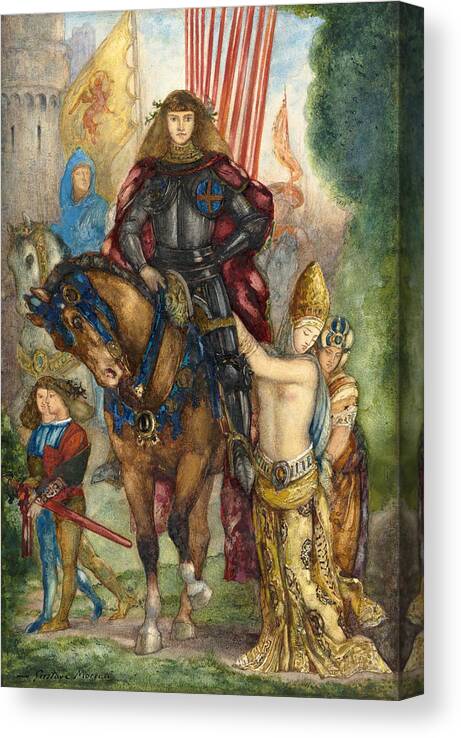This detailed Medieval-era painting, rendered on a slight 3D-effect rectangular canvas approximately five inches high and three inches wide, features a central scene dominated by a nobleman in gray armor with a flowing red cape, astride a majestic brown horse. The rider, with a laurel wreath crowning his long brown hair, commands attention with blue accoutrements embellishing his steed's bridle and reins. To the immediate right of the horse, a rather feminine figure with a Caucasian complexion is clad in a yellow skirt and wide white belt, while their head is adorned with a long, cylindrical yellow hat secured by a scarf under the chin.

Flanking the central duo, the scene is populated with various figures and elements that enhance the narrative and background. On the ground to the right, several people garbed in yellow clothes display somber expressions. Behind and slightly to the left, two children walk, juxtaposed by additional soldiers, regally carrying yellow flags adorned with possibly reddish dragon or horse motifs. Further in the background, another rider on a white horse is visible.

The setting captures aspects of a Medieval landscape, with a partially visible light brown castle on the left side and lush green tree tops and a brown rock resembling a face on the upper right side. The ground is covered in verdant grass under a clear blue sky, compiling to create an intricate and vibrant portrayal of the historical scene.